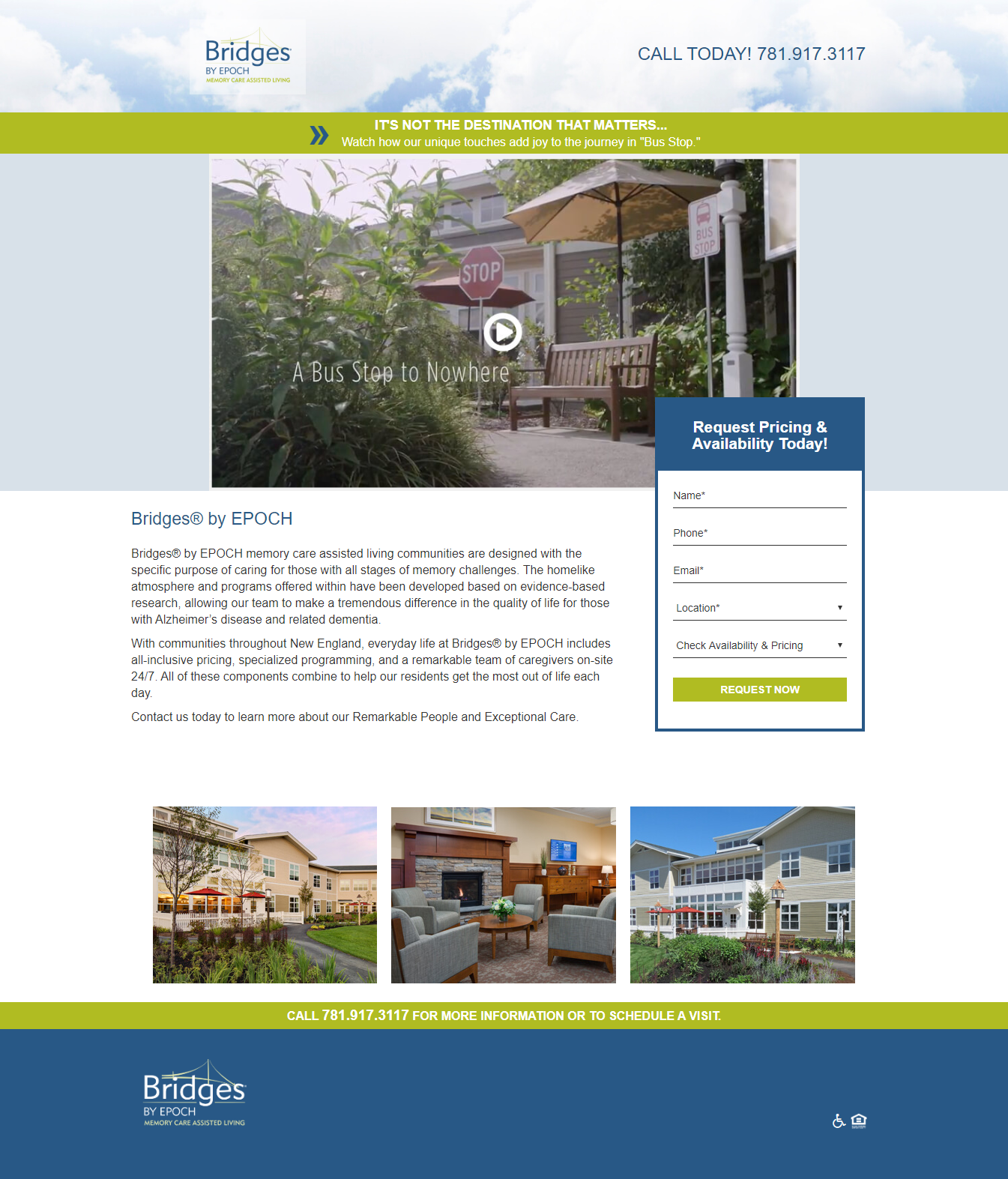The image features a vertically-oriented website layout. At the top, the background depicts a serene sky with fluffy white clouds. Towards the left side of this section, there is a translucent white rectangular area displaying the text "Bridges by Epcot." On the right side of this top section, a contact number "Call today: 781-917-3117" is prominently displayed.

Beneath, a green banner stretches across the width of the site, bearing the inspirational message: "It's not the destination that matters," accompanied by a double blue arrow at the front of the phrase. Below this banner, there is a more rectangular section flanked by light blue on the sides.

This section appears almost square and contains a photograph depicting a picturesque sidewalk scene. Elements in the photo include bushes on the left side, a bus stop sign, a pole that seems to be a light post, a bench, two large umbrellas, a tree, a building in the background, and a stop sign. The text "Bridges by Epcot" is located near this image, presumably to describe the illustrated area.

To the right of this section, there is a vertical rectangular area with a call-to-action: "Request pricing and availability today." This form requests the viewer's name, phone number, email, and location, with buttons to "Check Availability and Pricing" and "Request Now."

Below these interactive elements, there are three side-by-side pictures that suggest it's a community, likely apartments or homes. Confirming this assumption, it becomes clear that the website is for a "sustained living community." Additionally, a thin green banner below this section provides another contact number for further information.

Finally, a blue banner or border area at the bottom of the page reiterates the name "Bridges by Epcot" on the left side.